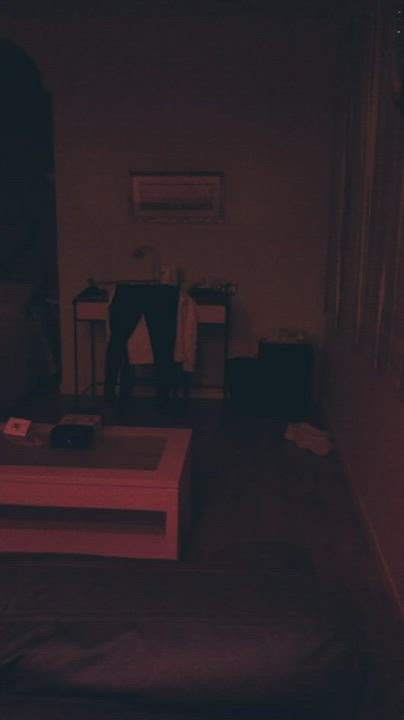A cozy room is dimly lit, suggesting the presence of a single lamp. Dominating the scene is a gray couch, positioned against a wall with white paint. Beside the couch stands a wooden end table adorned with various items. The flooring is wooden, enhancing the warmth of the room. To the side, there is a utility cart on wheels, doubling as a makeshift desk. On the cart, a lamp illuminates the surroundings, and a few pieces of clothing are casually draped over the chair that is pushed under it; a pair of pants and a shirt can be prominently seen. Nearby, a pair of shoes is placed neatly on the floor, and a black trash can sits discreetly in the background, adding to the lived-in feel of the space.